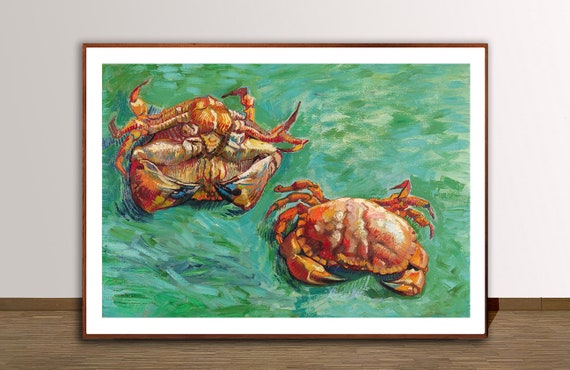This photograph showcases a detailed painting of two crabs, presented in a simple, thin brown frame with a white mat. The painting rests on a wooden surface against a white wall. The crabs are set against a swirly background of greens and blues, suggesting their natural, watery habitat. The crab on the top left is larger and more prominently depicted; it is primarily brown or orange, with claws and a visible mouth that some say resemble a human face. This crab appears to be in motion, its legs extended as if swimming. The crab on the bottom right is slightly smaller, facing downwards with its claws and legs tucked close to its body, showing off its red shell with black-tipped pincers. The vibrant brush strokes and lively depiction of the crabs create a bright and happy scene that captures the essence of their dynamic environment.